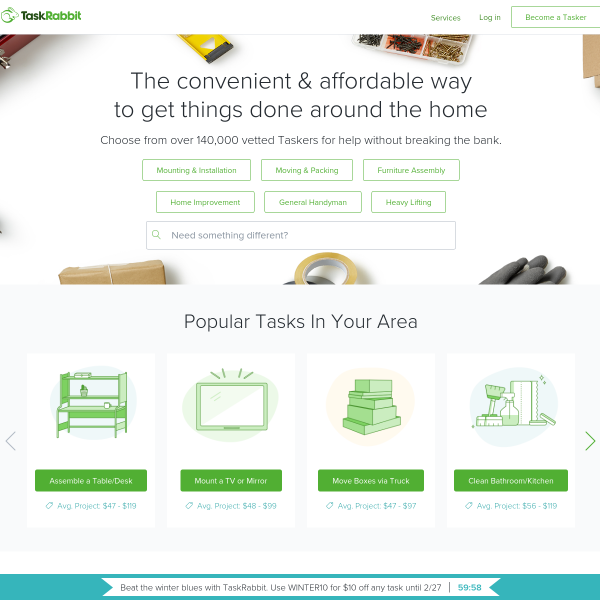**Descriptive Caption for TaskRabbit Webpage Screenshot**

The screenshot captures the landing page of TaskRabbit, which is roughly square-shaped and features a clean, white background. The header at the top contains the TaskRabbit logo on the upper left—depicting a curled green rabbit beside the text "TaskRabbit." The word "Task" is in a dark green hue while "Rabbit" is in medium green, both starting with capital letters. 

On the far right of the header, there are three clickable sections in green font: "Services," "Login," and "Become a Tasker." The "Become a Tasker" section is enclosed in a green box, suggesting it's a prominent call-to-action.

The main body of the webpage is dominated by a top-down image of a white table surrounded by various items: a roll of tape at the bottom center, the fingers of work gloves at the bottom right, a wrapped cardboard box at the bottom left, an indistinguishable item at the top center, and a sectioned storage container at the top right filled with small objects like nails.

Centered in the middle of the page, a large, dark gray text reads: “The convenient & affordable way to get things done around the home.” Beneath it, in smaller font, it says: “Choose from over 140,000 vetted Taskers for help without breaking the bank,” with “Taskers” capitalized.

Directly below this slogan are two rows of three green-outlined boxes, each containing specific services: 
1. Mounting & Installation
2. Home Improvement

Below these service categories is a centrally aligned, long search field with a gray outline. It features a magnifying glass icon on the left and the text, “Need something different?”

The lower section of the webpage has a light gray background and is titled "Popular Tasks in Your Area,” with each word capitalized. This section includes four illustration-based clickable sections, all with green and white color schemes:
1. A desk assembly task is represented by a desk with shelves illustration, with a clickable green field below saying, “Assemble a Table/Desk” and an average project cost of $47-$119 in light blue text.
2. A TV monitor illustration for mounting tasks reads “Mount a TV or Mirror,” with an average project cost of $48-$99.
3. A stack of boxes illustration labeled “Move Boxes via Truck,” showing an average project cost of $47-$97.
4. Cleaning supplies illustration reading “Clean Bathroom/Kitchen,” with an average project cost of $56-$119.

To navigate these options, arrowheads are displayed to the left and right of the four tasks.

At the very bottom, a medium teal box spans the width of the page. This box contains a white search field with a promotional message in black font: “Beat the winter blues with TaskRabbit.” It offers a discount code, WINTER10, for $10 off any task until February 27, alongside a countdown timer.

Overall, the webpage is visually organized, user-friendly, and efficiently designed to promote their wide range of services and encourage user interaction.